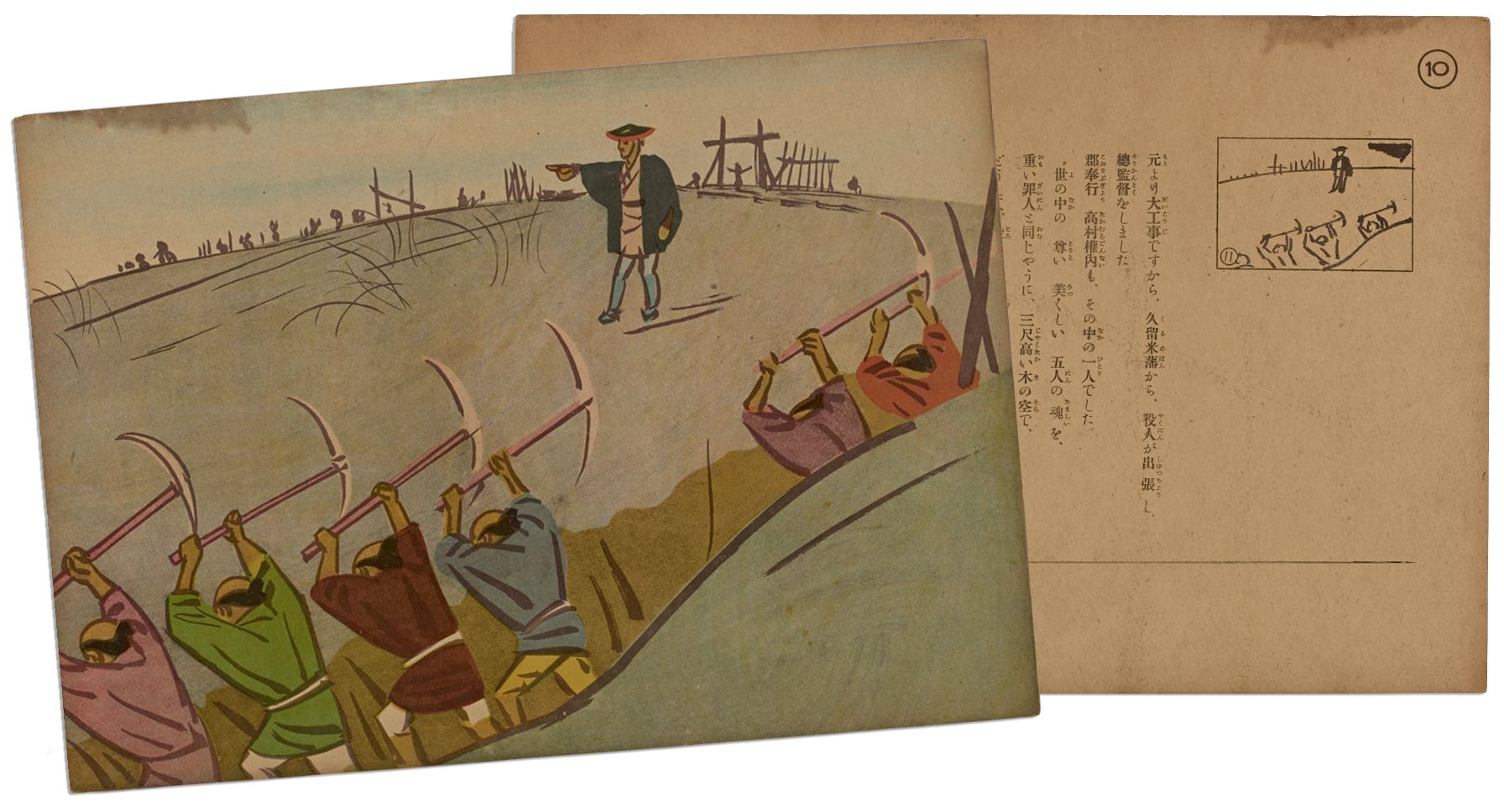The image is a detailed drawing that seems to depict both the front and back of a postcard. On the left side, a man dressed as a traditional Japanese leader points to the left, wearing a distinctive triangular hat and a green cap. To his left, six men, adorned in colorful outfits—pink, green, brown, blue, purple, and red—are engaged in intense digging with hoes, standing in what appears to be a ditch. This side also features a smaller depiction of the main image, enclosed in a rectangular box, and a brown piece of paper with Japanese text. The right side of the image includes the Japanese text aligned vertically, topped with a circled number '10' in black. The composition captures a snapshot reminiscent of historical or commemorative artwork, blending traditional clothing with the labor scene, possibly reflecting a specific historical or cultural narrative.